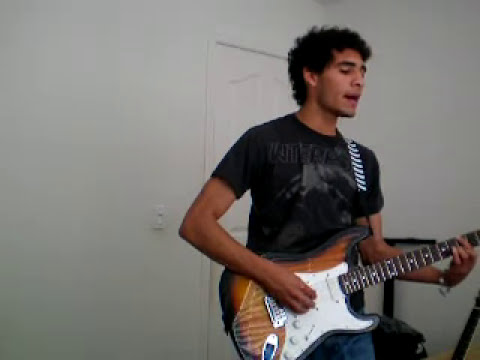In the image, a young man with curly black hair and a tan complexion is passionately playing an electric guitar in a room with white walls. He's positioned at an angle, facing the right side, with a white door and a modern light switch in the background. His eyes are partially closed, and his mouth is slightly open, suggesting he's singing or deeply immersed in his music. He's wearing a black t-shirt featuring a light grey graphic, possibly of a band like Pantera, and jeans. The guitar has a glossy wood trim and a white panel on the lower part, with various knobs. He grips the guitar's neck with one hand, while strumming near the base strings with the other. A black and white striped guitar strap is slung over his left shoulder. The image captures the intensity and focus of his performance, highlighting his connection to the music.